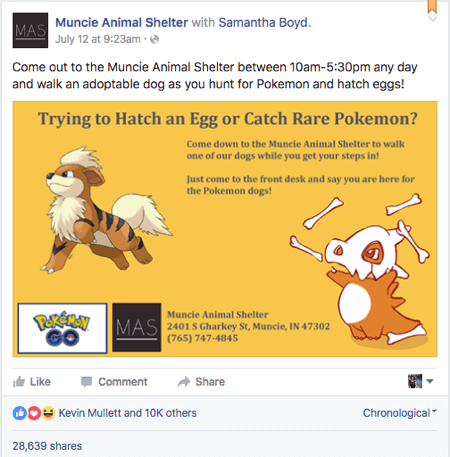Join us at the Muncie Animal Shelter for a fun-filled day of dog walking and Pokémon hunting with Samantha Boyd! From 10 a.m. to 5:30 p.m. daily, you can walk an adoptable dog while searching for Pokémon and hatching eggs. This unique experience not only gives these lovable dogs some much-needed exercise but also adds an exciting twist to your Pokémon Go adventures. The announcement, made on July 12th at 9:23 a.m., features a playful image of a dog alongside Pokémon-themed graphics, inviting everyone to "hatch an egg or catch rare Pokémon." Don't miss out on this paw-some opportunity to combine your love for animals and gaming! Come to the Muncie Animal Shelter and enjoy seven and a half hours of canine fun every day.